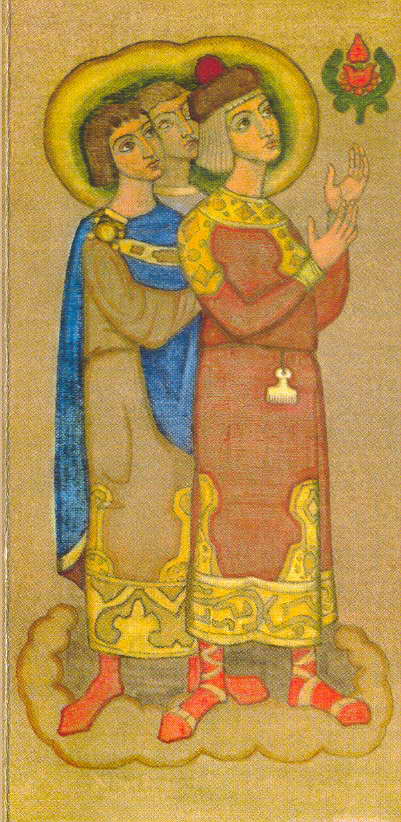The image depicts a medieval-style portrait of three individuals adorned in ornate robes and accessories. They appear to be standing, with two figures in the foreground and one slightly behind. The figure on the left is attired in a blue and tannish robe with gold accents, while the figure on the right dons a red robe with similar gold detailing. Both are wearing red socks, though one has an additional pattern with white zigzags. The individual on the right raises their hands slightly as if gesturing towards a floating green emblem with a red insignia, possibly a symbol or a candle holder, situated in the upper right corner. One of the figures in the portrait wears a hat resembling a beret with a red pouf on top, and all have pageboy haircuts. Behind them, there is a gold-bordered mirror reflecting one of the figures, and all three possess a singular halo encircling their heads, adding a religious aura to the scene. The intricate background and accessories, including a blue cape with a shoulder clasp and potential keys or combs at their waists, enhance the image's rich, historical ambiance.